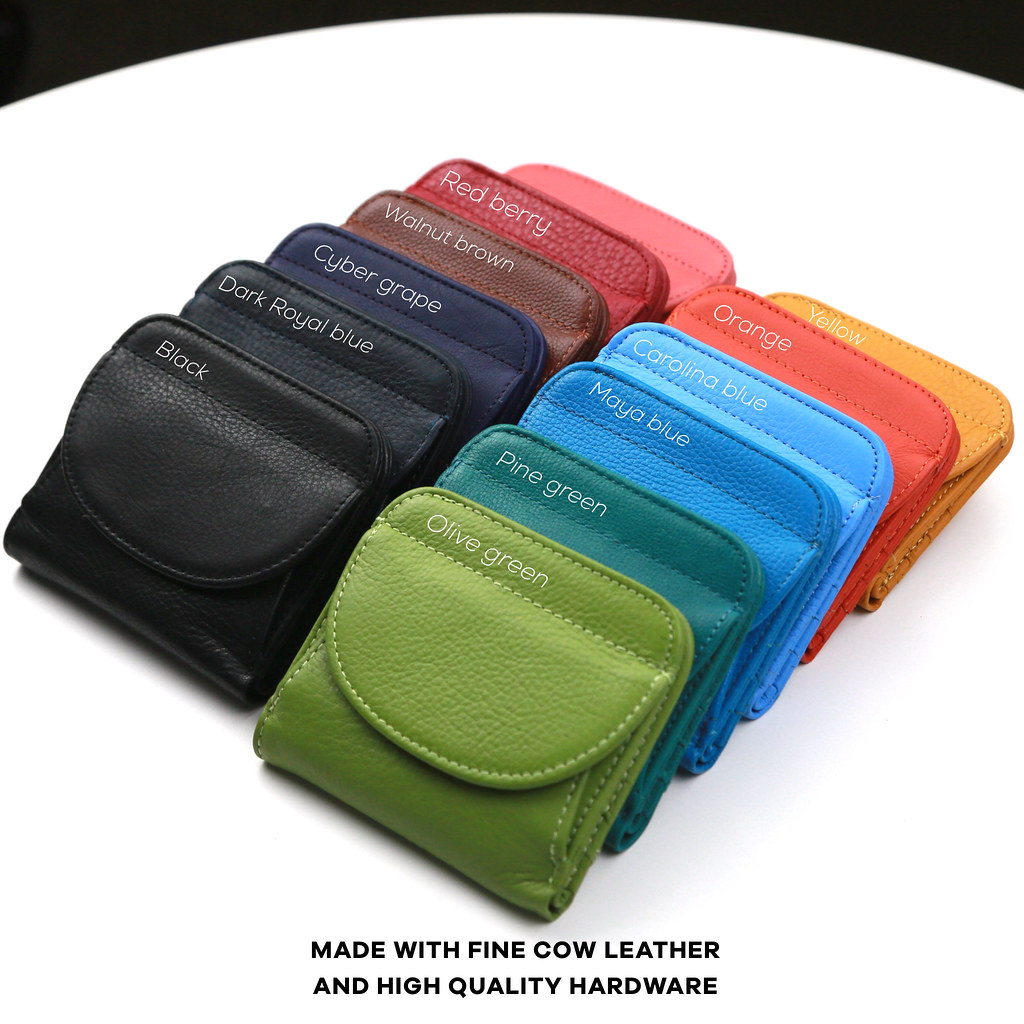The image showcases a detailed and vibrant advertisement for small, high-quality wallets crafted from fine cow leather and high-quality hardware. The wallets are neatly arranged in two rows, with one row stacked behind the other, displayed on a clean white circular background with a subtly curved black border at the top. Emphasizing their exquisite craftsmanship, the bottom of the image features the text "Made with fine cow leather and high quality hardware" in black letters.

Each wallet is adorned with unique colors, and their respective names are typed in white font directly on them. The wallets start with an olive green and a pine green, followed by a Maya blue and a Carolina blue. In addition, vibrant shades include an orange, a yellow that resembles mustard, a classic black, a dark royal blue that appears almost blackish-blue, and a cyber grape color, which looks like a dark blue with hints of purple. Further variety is presented with a walnut brown, a red berry, and finally, a pink wallet, though partially fallen and unlabeled, adds a unique touch to the assortment. Each wallet maintains a consistent style with some stitched in contrasting colors, highlighting the meticulous attention to detail of the design.